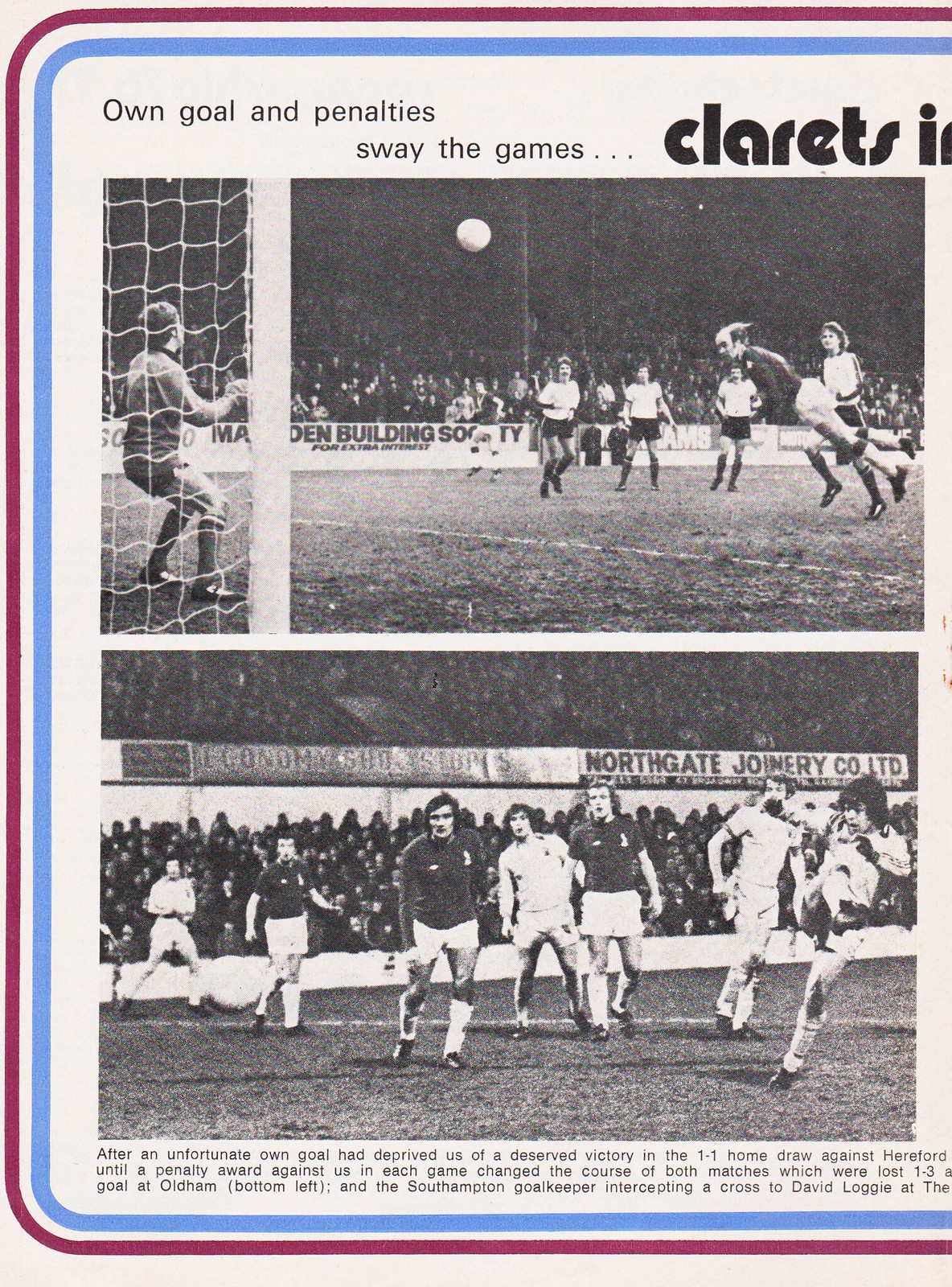The image depicts a vintage football program page, showcasing two black-and-white action photographs framed within a maroon, light blue, and white triple border. At the top left corner, the text starts with "Own goal and penalties sway the games..." in small black font. Below this, in large capital letters, is the partially visible word "CLARETS IN." The top photograph features a dynamic scene with a player suspended mid-air, appearing to have just headed the ball towards the goal being defended by a keeper, with several other players in white kits and black shorts also engaged in the play. The lower photograph shows additional players in black and white uniforms on the field, facing the viewer, with a crowded audience visible in the backdrop. There’s noticeable signage on a banner reading "Northgate Joinery Co. Ltd." Text beneath the photos provides narrative but is cut off, starting with "After an unfortunate goal had deprived us of a deserved victory in the 1-1 home draw against Hereford," and continues fragmented with details about penalties and match outcomes. The page, likely part of a broader two-page spread, captures the momentum and atmosphere of a historic football match.